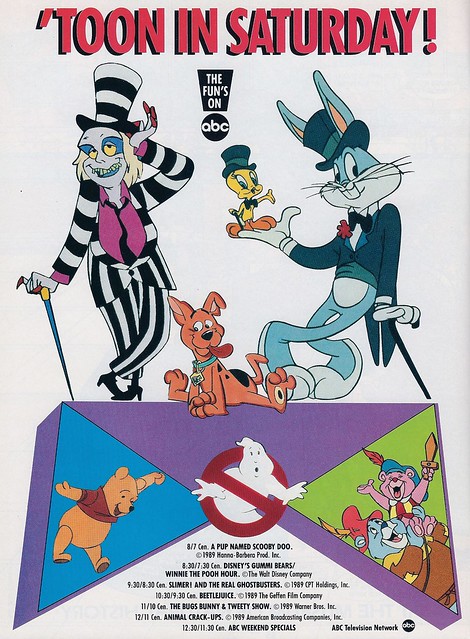This image is an advertisement for a Saturday morning cartoon block on ABC television network, designed to appeal to fans of various animated series. At the top, bold red text with an exclamation mark reads, "Tune in Saturday T-O-O-N," touting the fun lineup with the message, "The fun's on ABC." The image showcases a range of beloved characters: on the left, Beetlejuice in his signature black-and-white suit and pink shirt, resting on a cane; in the center, the younger Scooby-Doo from "A Pup Named Scooby-Doo"; and on the right, a dapper Bugs Bunny in a tuxedo and top hat, holding Tweety Bird who is similarly dressed with a top hat, bow tie, and cane. 

Below these characters, the image is divided into colorful triangles containing more cartoon favorites. On the bottom left is Winnie the Pooh, while adjacent is the Ghostbusters symbol. The bottom right features two Gummy Bears in medieval garb: a pink child bear holding a wooden sword and a blue adult bear. Beneath these segments, a schedule lists the airing times for the shows, set against a vibrant backdrop of purples, blues, and greens, giving the entire ad a lively and playful feel.